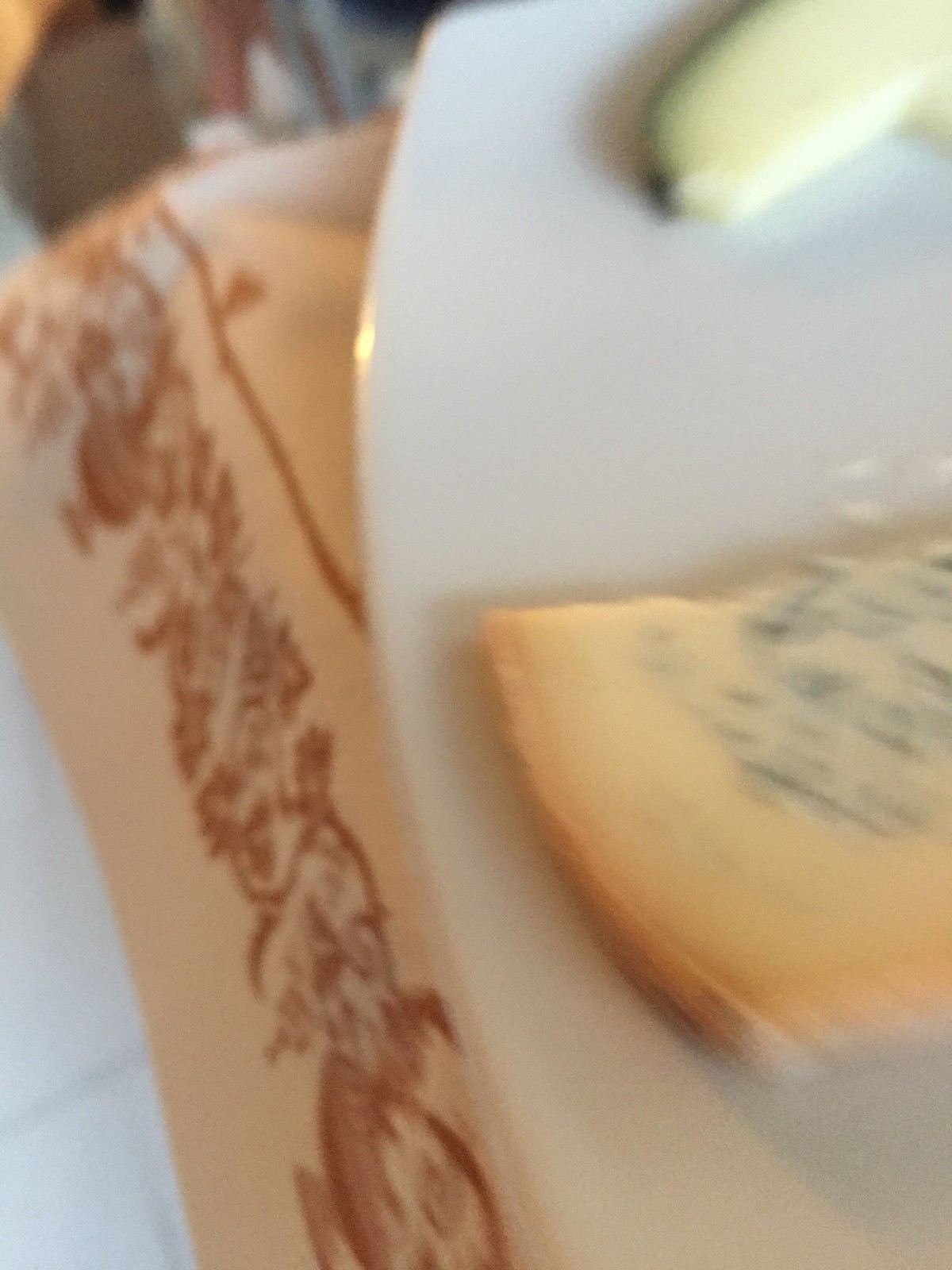In this out-of-focus and blurry color photograph taken in portrait mode, we see a close-up of a white ceramic plate adorned with a gold trim, partially captured in the frame. The plate rests on what seems to be a tan or cream-colored decorative fabric featuring ornate, vine-like brown designs, possibly resembling Italian motifs with vases and intricate details. On the upper side of the plate, there appears to be a greenish-white object with a dark green edge, likely a fruit or a pickle spear showing only the rind. Toward the bottom of the plate, an orange-yellow item with gray specks in the middle can be seen; it might be a slice of cheese, such as blue cheese with its characteristic mold flecks, or even a piece of cantaloupe. The table under the decorative fabric, partially visible, seems to be white.